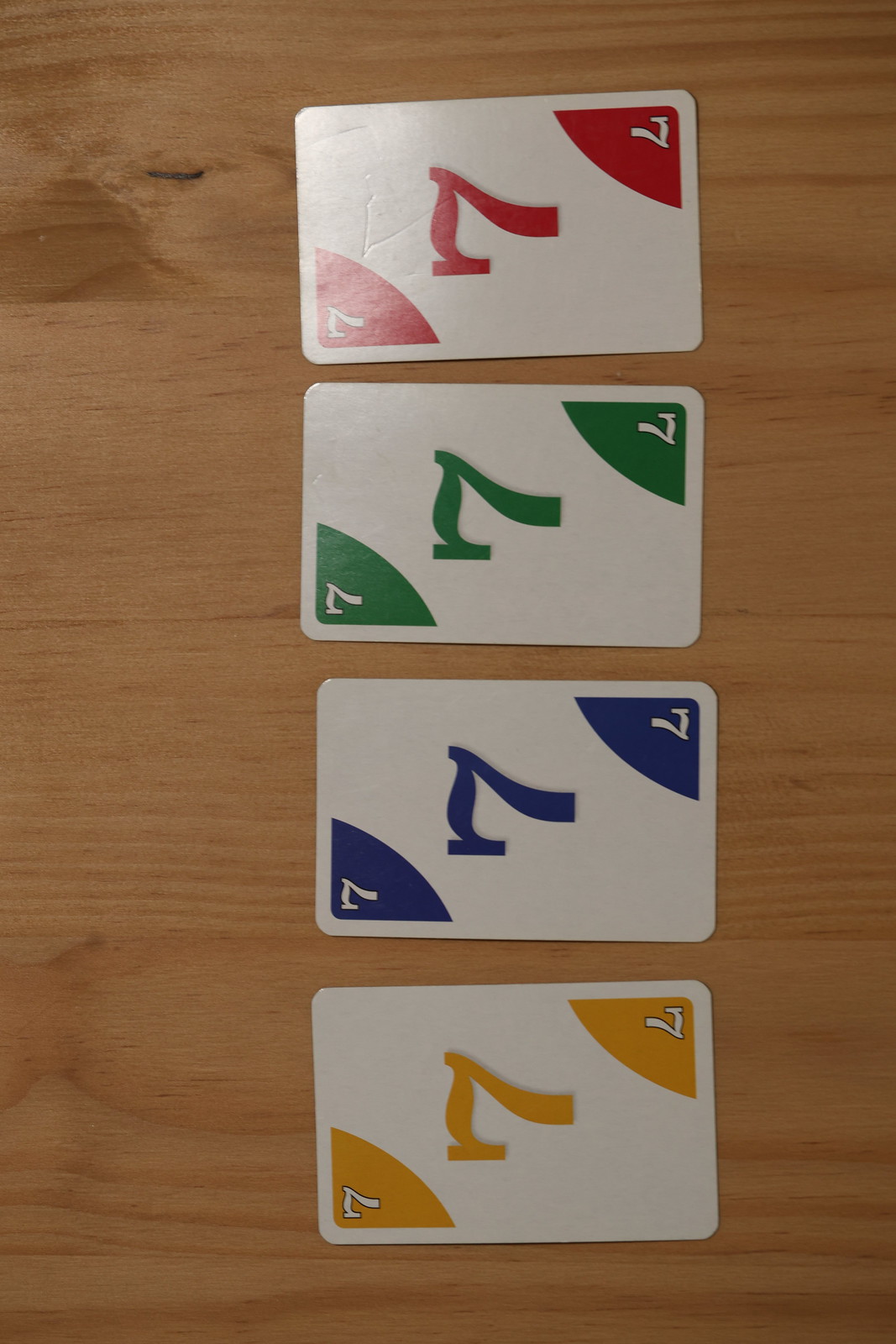The image depicts four Uno cards, each featuring the number seven, arranged vertically with all cards turned sideways. The cards are displayed in a sequence of colors from top to bottom: red, green, blue, and yellow. Each large number seven is prominently colored to match the card's background, and smaller sevens can be found in the top left and bottom right corners of each card, designed with a similar triangular pattern background. Notably, the red card at the top shows visible signs of wear, including scratch marks and dents.